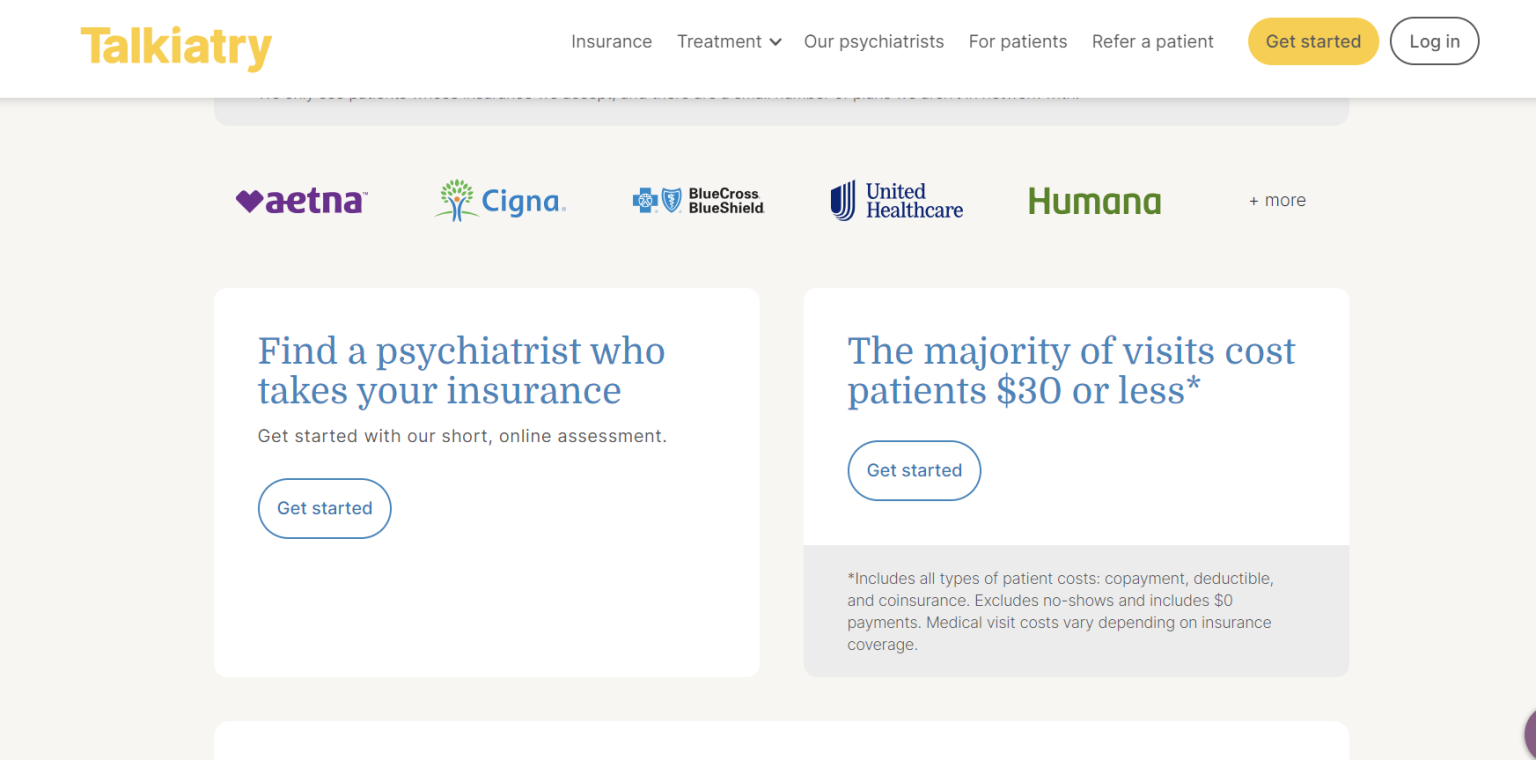This is an image from the website Talkiatry. At the very top, the word "Talkiatry" is displayed in bold yellow font against a white background. The header contains several navigation options, also set against this white background, including "Insurance," "Treatment," "Our Psychiatrists," "For Patients," "Refer a Patient." Additionally, there is a prominent yellow button labeled "Get Started," alongside a white "Log In" button.

Below the header, the background shifts to light gray. Featured prominently are logos of well-known insurance companies, including Aetna, Cigna, Blue Cross Blue Shield, United Healthcare, Humana, and a label indicating "plus more."

On this light gray background, there are two white rectangular sections. The left rectangle invites visitors to "Find a psychiatrist who takes your insurance," and promotes taking a "short online assessment" with a "Get Started" button. The right rectangle informs visitors that "The majority of visits cost patients thirty dollars or less," and also includes a "Get Started" button. Below these sections is some fine print and a gray box at the very bottom of the image.